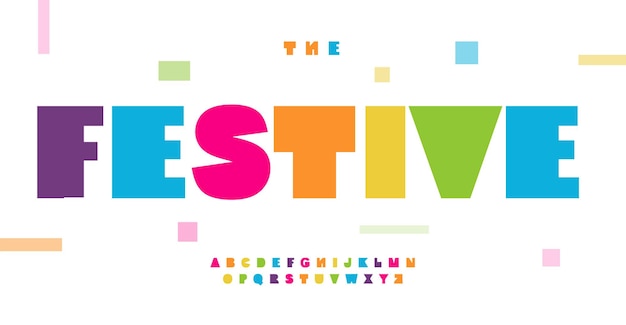The image showcases a vibrant, festive-themed graphic with a clean white background. At the top, in smaller text, it reads “the” with "th" in orange and "e" in blue. Dominating the center is the word “festive” in bold, rainbow-colored letters: F in purple, E in blue, S in bright pink, T in orange, I in yellow, V in green, and E in blue again. Surrounding the word “festive” are small pastel colored squares and rectangles in hues of yellow, blue, green, and pink, giving a confetti-like appearance. At the bottom, the entire alphabet is displayed in a repeating rainbow pattern from pink to purple. The overall design emphasizes a unique and playful typeface with multi-colored and varied shapes throughout the graphic.